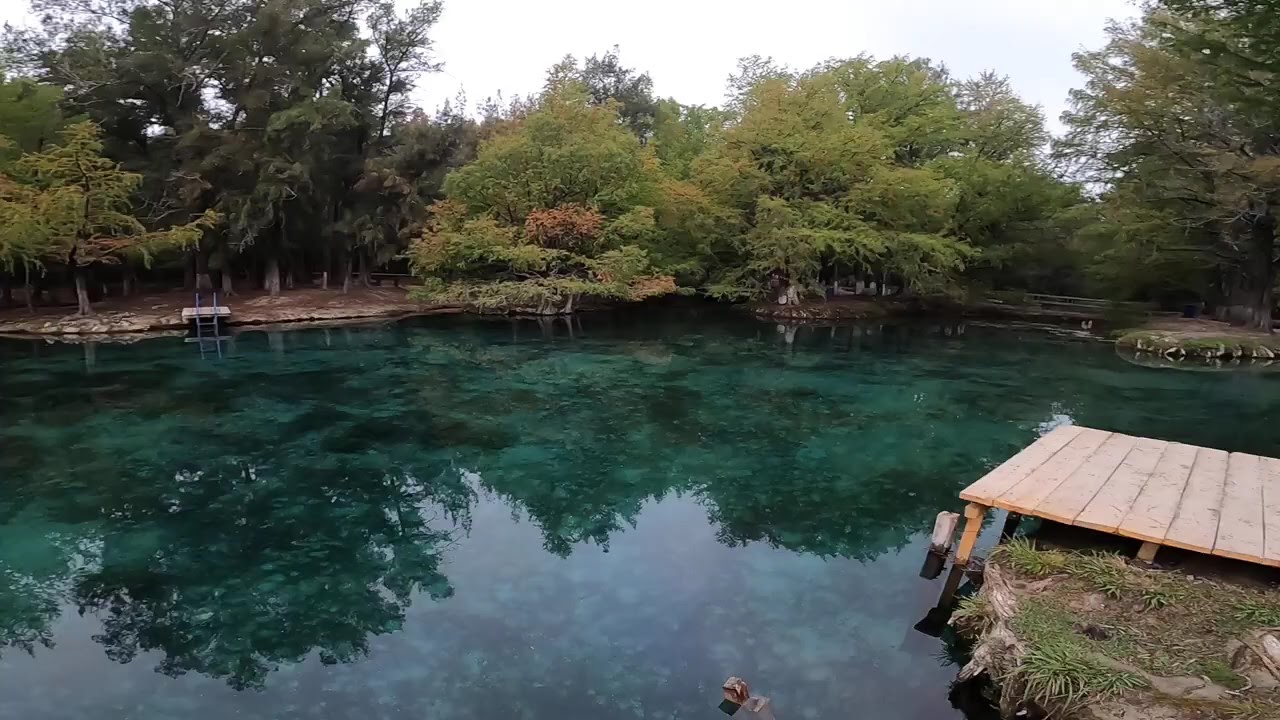The image captures a private vacation spot featuring a serene, turquoise-green pond. The crystal-clear, still water beautifully reflects the surrounding environment, including lush green trees on the opposite shore, some interspersed with touches of orange foliage. The sky above is a gradient from light blue to white. In the foreground, a small wooden dock juts out from the bottom right corner, extending only a short distance into the reflective water. There is a patch of grass and dirt land near the dock. On the far side of the pond, the shore curves gently, populated with large, fluffy trees that appear to grow out of the water. White spots in the water, possibly rocks, add texture to the scene. A rocky beach area and another dock with a ladder can be spotted in the background, augmenting the picturesque setting.